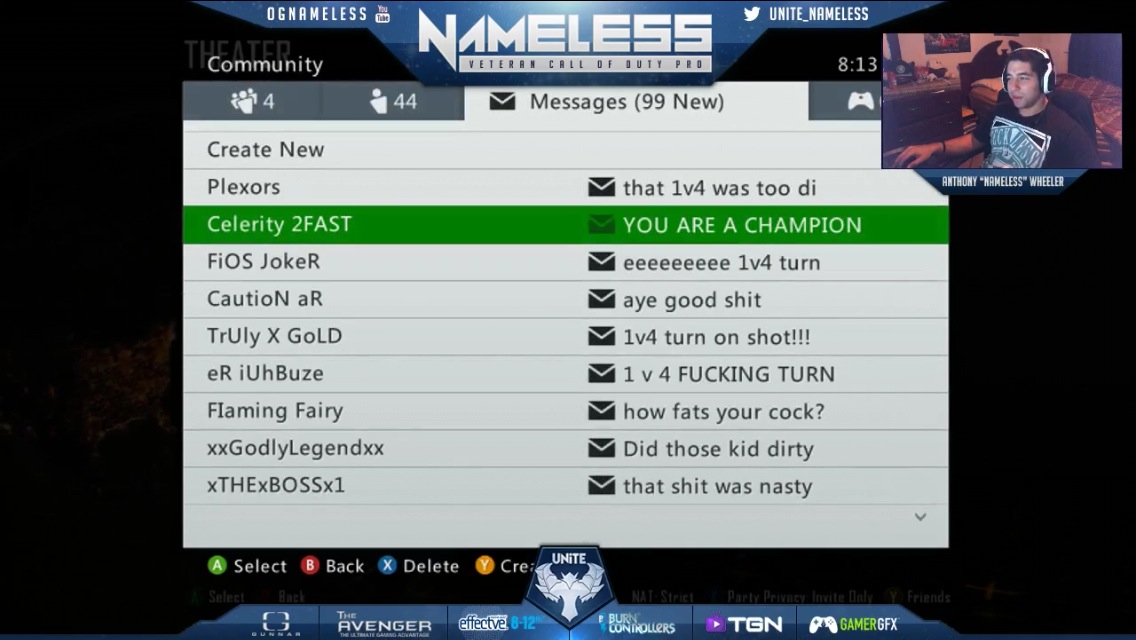The screenshot image depicts a gaming interface, presumably from Xbox, with the username "OGNAMELESS" prominently displayed in the top left corner, while "Veteran Call of Duty Pro" is labelled beneath "NAMELESS" in the middle. In the top right, there is a Twitter icon accompanied by the handle "UNITE_NAMELESS" and the timestamp "8:13." The left-hand side of the screen features a menu with "COMMUNITY" and the highlighted option "MESSAGES," indicating "99NEW" messages. Notable messages include ones from users such as Plexors, Celerity2FAST, Fios Joker, CautionAR, TrulyXGold, ERIUH Boozey, FlamingFairy, XXGodlyLegendXX, and XVXBossX1. Among the messages, a highlighted one from "Celerity2FAST" reads "YOU ARE A CHAMPION." Interface commands displayed on the bottom left include "A for SELECT," "B for BACK," "X for DELETE," and "Y for CREATE." Additionally, the top-right corner of the screenshot shows an inset image of a person wearing headphones, seated with a bed and chest of drawers in the background, suggesting a casual gaming environment.